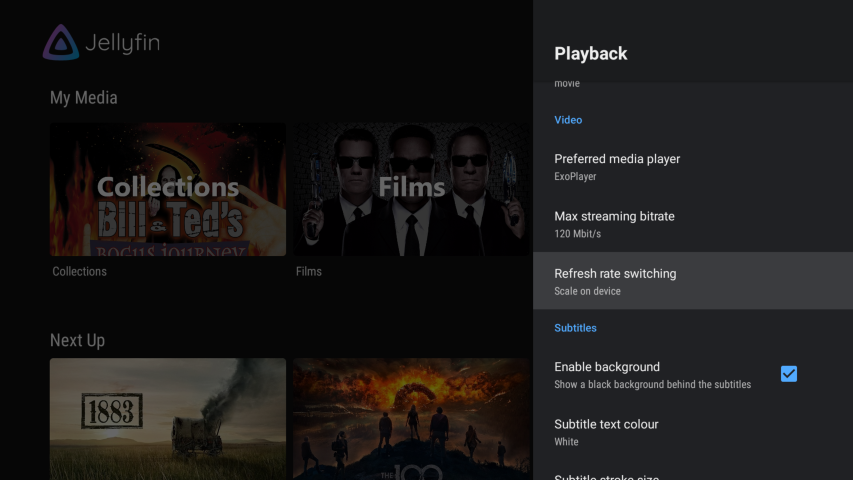This is a detailed screenshot of a media player interface, predominantly featuring dark gray and black tones. The main screen is semi-opaque due to an open navigation panel on the right-hand side.

In the top left corner of the main screen, there's a multicolored triangle logo with a smaller triangle inside it, accompanied by the text "Jellyfin". Below this, "My Media" is prominently displayed in white font. The screen is sectioned into rows showcasing different media categories.

The first category, labeled "Collections," features an image from "Bill and Ted's Excellent Adventure" as its display image. To the right, the "Films" section displays the cover image for "Men in Black."

In the second row, the "Next Up" section includes the TV series "1883" from "Yellowstone", with the show "The 100" next to it on the right.

On the navigation panel to the right, several playback settings are listed:
- "Play Back" or potentially "Playback."
- "Movie" and "Video" options.
- "Preferred Media Player" set to ExoPlayer.
- "Max Streaming Bitrate" configured to 120 megabits per second.
- Settings like "Refresh Rate Switching" and "Scale on Device."
- Subtitles settings with an enabled option for "Show a black background behind the subtitles," which is ticked Yes, indicating it’s activated. The subtitle text color is set to white.

This organized layout and detailed options provide users with a customizable and user-friendly media experience.